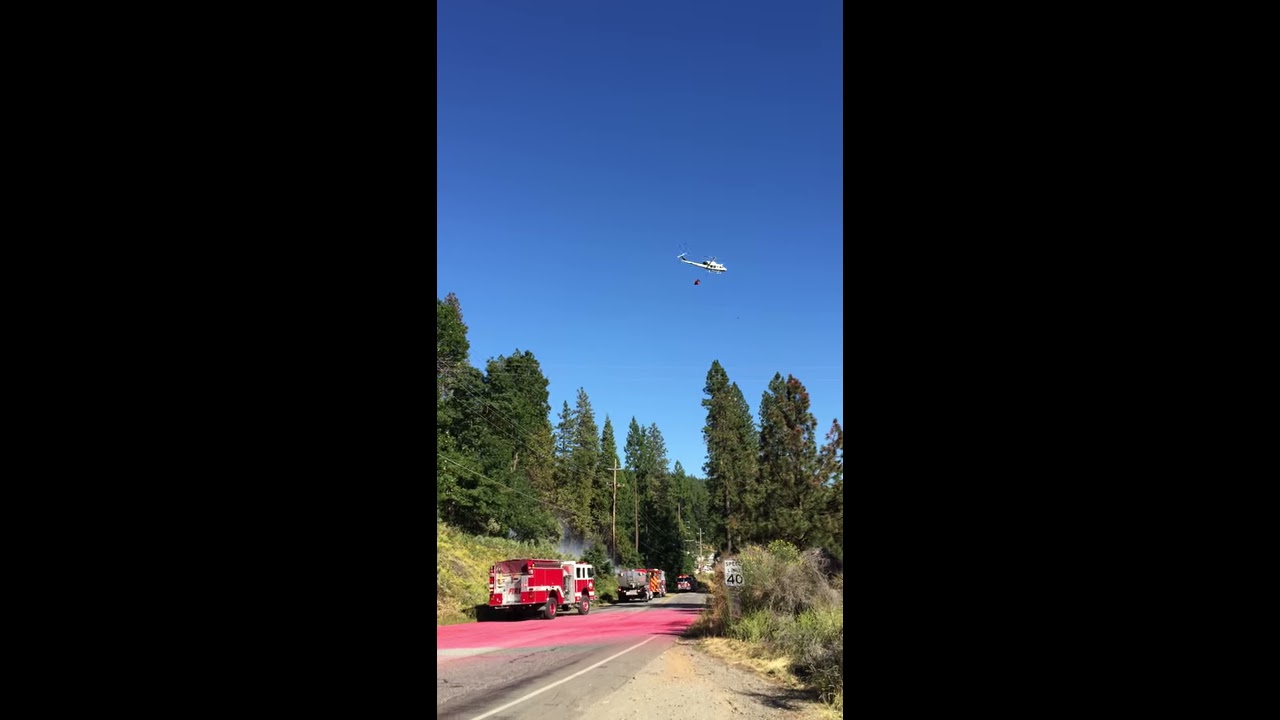In this detailed image, we see a forest landscape dominated by tall green pine trees and dense shrubbery, set beneath a clear, sunny midday sky. A major focus is a white helicopter hovering mid-air, carrying a red cylinder object, likely a water barrel used to combat the forest fire implied by the visible smoke in the background. Below, a mountain road angles upward, featuring three red and white fire trucks, some with yellow and gray markings, signifying the active presence of a fire rescue team. The road itself, partially covered with what appears to be red fire retardant powder, meanders through the scene with surrounding grassy areas and various bushes. Adjacent to this road, utility poles with power lines run along the embankment, alongside a prominent speed limit sign reading "40 mph" in black text. Off in the distance, possibly the edge of a town can be inferred. The left side of the image includes a concrete pathway or parking area connecting to the main road. The overall setting conveys a tense yet organized emergency response in a tranquil rural forest area.